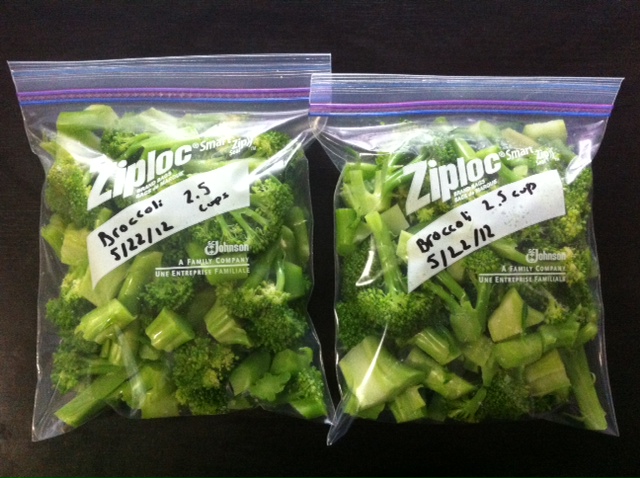This image captures two clear Ziploc bags filled with diced broccoli pieces, each positioned against a solid black background. Both bags prominently showcase the brand name “Ziploc” in white lettering along the top, specifically indicating “Ziploc Smart Zip.” Each bag features a distinguishable closure with a combined purple and blue stripe, visually marking where the bags have been sealed. Beneath the Ziploc logo, there is a white writable label where someone has inscribed “broccoli, 2.5 cups” followed by the date “5/22/12” in black ink. Additionally, both bags also display the text “Johnson, a family company” indicating the manufacturer. The uniform presentation suggests the broccoli is prepped and ready for either freezing or refrigeration.